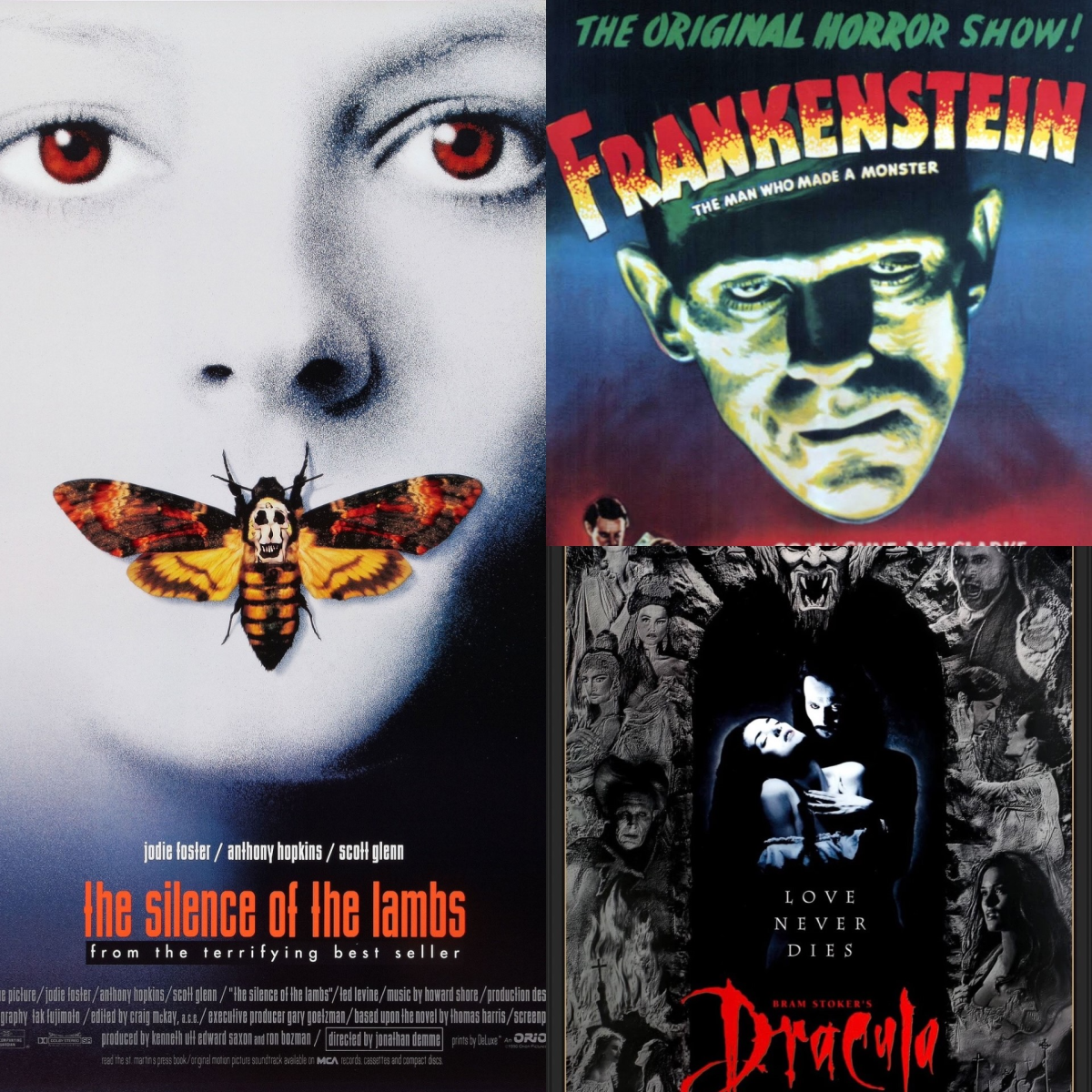This advertisement, likely a promotional poster for a theater's double or triple feature, vividly combines elements from three classic horror movies: "The Silence of the Lambs," "Frankenstein," and "Dracula." On the left side, a striking "The Silence of the Lambs" poster dominates, featuring a close-up of a woman’s white face with red eyes, her mouth obscured by a butterfly whose wings resemble flames and bear a small skull. The movie title is prominently displayed in orange letters, with actors' names—Jodie Foster, Anthony Hopkins, and Scott Glenn—listed above, along with the tagline, "From the terrifying bestseller."

On the right side, the upper half is dedicated to "Frankenstein," with the title in fiery red and yellow letters under a green banner reading "The Original Horror Show." The image showcases the monster's face with green skin and a towering forehead. Below, the section for "Dracula" features the title in bold, bloody red letters. It displays a menacing man, potentially Bram Stoker's Dracula, holding a woman, possibly Winona Ryder’s character, surrounded by a dark, eerie ambiance with gray-toned figures collaged around them. The tagline "Love Never Dies" is ominously included to emphasize the gothic romance element. This detailed and colorful artwork masterfully intertwines the macabre essence of each classic film.